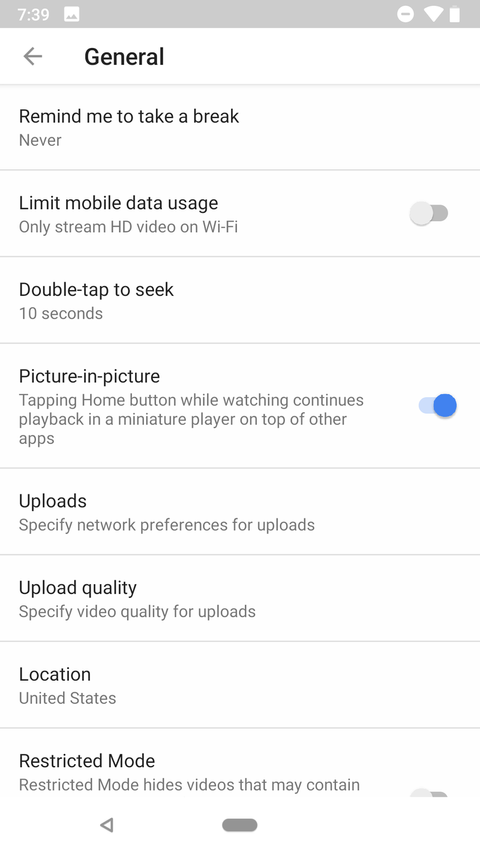This image depicts a screenshot taken from a cell phone interface. Recognizable cell phone icons are visible in the top corners of the screen, with the upper right displaying the battery icon, Wi-Fi icon, and a Do Not Disturb icon (circle with a horizontal line through it). Under these icons, the content begins with the title "General."

The first option listed under "General" is "Remind me to take a break," which is currently not selected. Following this, the section titled "Limit mobile data usage" features a sub-option "Only stream high definition video on Wi-Fi," which is toggled off.

Further down, the setting "Double-tap to seek" is set to 10 seconds. Directly beneath this, the "Picture-in-picture" feature is highlighted and is toggled on.

The next segment, labeled "Uploads," provides specified network preferences for uploads and includes an option for "Upload quality" to specify video quality for uploads. Finally, the location setting indicates that it is set to "United States."